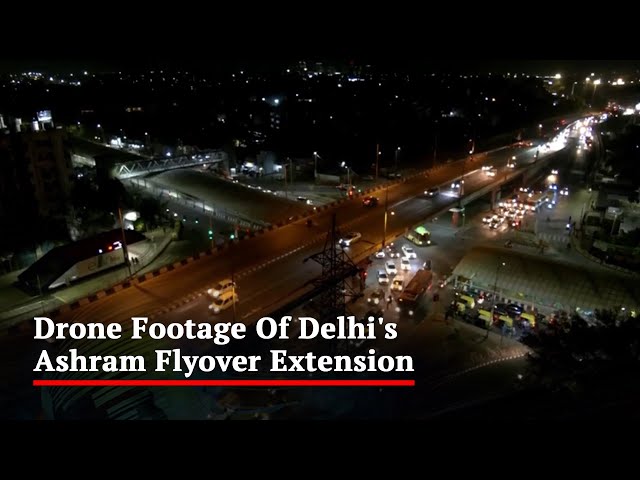This nighttime aerial photograph showcases the bustling Ashram Flyover Extension in Delhi, India, captured via drone. The image features a complex highway intersection where an elevated, long overpass supported by pylons runs above another highway that intersects it at a T. Below the elevated highway, a third roadway parallels it. At the dead end of the T, there stands a distinctive large building with glass panels, resembling a Quonset hut. The photograph is filled with the illumination of numerous vehicles' headlights, especially noticeable as they navigate the T intersection toward the camera. The backdrop reveals a vibrant cityscape dotted with countless city lights against a stark black horizon. In the lower left-hand corner of the image, bold white text reads, "Drone footage of Delhi's Ashram Flyover Extension" with a horizontal red line beneath it, further emphasizing the clarity and modernity of the scene.